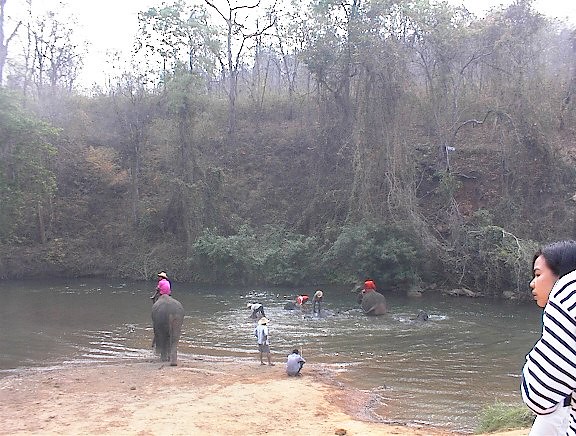The image is a realistic, horizontally-oriented nature scene photographed outdoors during the day under bright, light gray skies. Central to the scene is a body of water, likely a pond or lake, with a backdrop of a hill or bluff descending into the water, lined with trees, bushes, and grass. In the water, several people are seen, some wearing shirts and shorts, and others sporting hats. Notably, there are two elephants in the photo: one being ridden by a person in a red shirt located in the water, with the water reaching the elephant's legs, and another elephant on the sand to the left, ridden by someone in a pink shirt and straw hat. In the bottom left, a sandy beach area is visible with a couple of people standing. On the right, partially visible, a person with medium brown skin wearing a black and white striped shirt is either leaning or sitting. The distant background features tall trees and brush, providing a lush, natural setting above the river-like area where the activities are taking place.